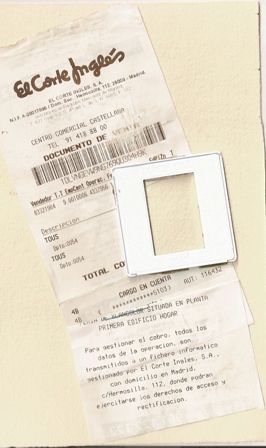This photograph features a receipt in Spanish from the store El Corte Inglés, set against a beige or off-white background. The receipt is angled approximately 30 degrees to the left and shows various details including a barcode, the store name, vendor information, descriptions of purchased items, and partially obscured total and checkout information. Notably, the last four digits of a credit card ending in 5103 are visible with the preceding numbers asterisked out. A unique element in the image is a small white frame, resembling a slide projector cutout. This frame is placed over the receipt about halfway down the image, with its opaque or translucent center seamlessly blending with the beige background, thereby partly hiding the receipt beneath. The bottom of the receipt appears folded, with some questions or text visible on the fold, contributing to the overall layered and slightly disorganized composition.